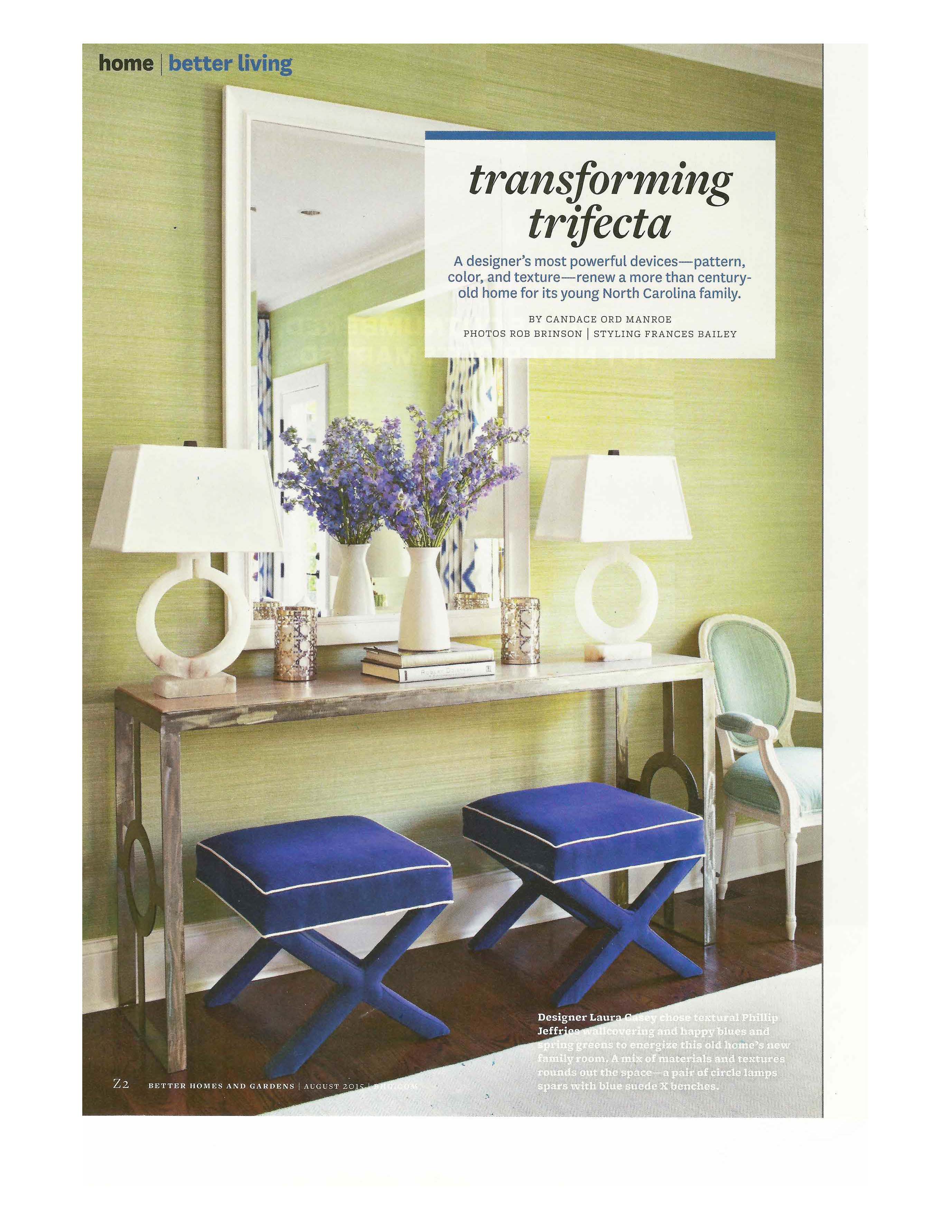Captured in an elegantly styled interior scene, this magazine page from "Home, Better Living" features a sophisticated vanity table set against a pale straw-green wall. Atop the table, which is flanked by two modern white lamps with square shades, stands a large mirror bordered by a vase of purple flowers positioned on a couple of neatly stacked books. Complementing the setup are ornamental cans, presumably silver or brass, adding a touch of elegance. Below the table, two stools with blue legs and cushions are neatly tucked in, while to the right, a green chair with a thick cushion rests against the rich, hardwood floor. The upper left-hand corner of the page prominently displays the magazine title, "Home, Better Living," and additional text across the top reads: "Transforming Trifecta: A Designer's Most Powerful Devices—Pattern, Color, and Texture Renew a More Than Century-Old Home for Its Young North Carolina Family," with credits to Candice Manor for writing, Bob Benson for photography, and Frances Bailey for styling. Additional brief text snippets adorn the corners, adding to the sophisticated aesthetic of the magazine layout.